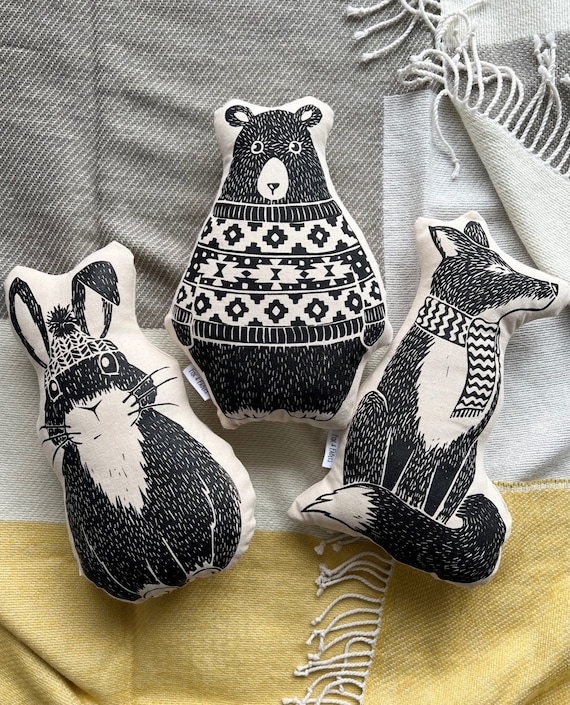This image features three black-and-white cloth characters intricately drawn on individual white pillows. The left pillow showcases a rabbit with a striped beanie hat, including a pom-pom, and one ear bent down. The middle pillow displays a bear adorned in a diamond-patterned sweater, with distinct detailing showing its fur, nose, eyes, and ears. The right pillow presents a fox wearing a striped scarf, with its closed eyes suggesting a peaceful demeanor. The characters rest on a layered fabric background, consisting of a gray blanket with white frayed edges, beneath which lies a beige-gold cloth also edged in white frills. The scene, seemingly taken inside a home, features a cozy arrangement that highlights the intricately designed pillows against the soft textile layers.